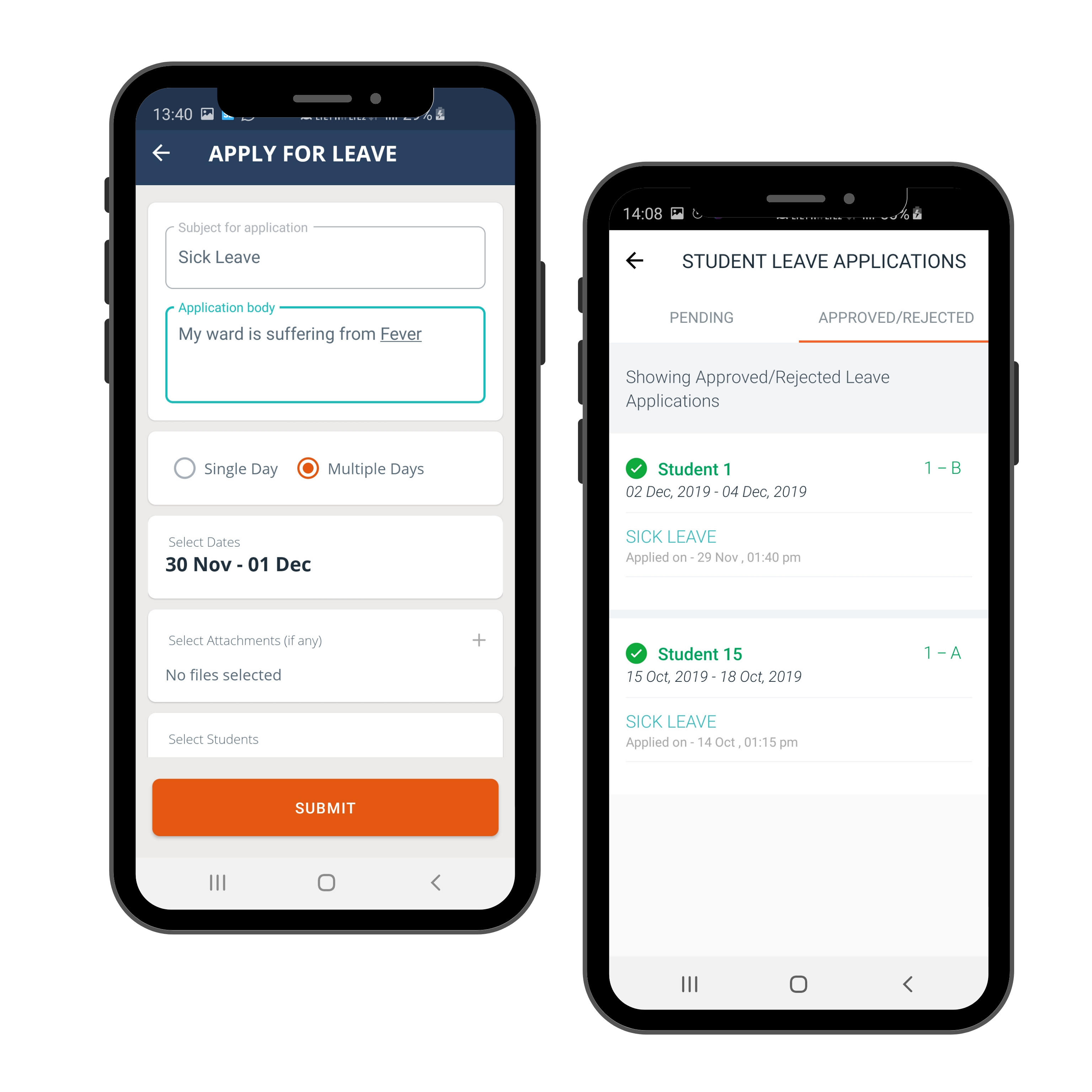The image features two smartphone screens side by side. 

On the left screen, you're presented with an interface designed for submitting a leave application. The top section is in dark blue, prominently displaying the text "APPLY FOR LEAVE" in white, capital letters. Below, fields are laid out for detailing the application: 

- **Subject for Application:** Sick Leave
- **Application Body:** "My ward is suffering from fever."

Below these text fields, the user is given a choice between two radio buttons: "Single Days" and "Multiple Days." The "Multiple Days" option is selected, indicated by a circle filled with orange. Further down, there are options to:

- **Select Dates:** From 30 November to 01 December
- **Select Attachments, if any:** Currently, it reads "No file selected."
- **Select Students:** (The specific options or details are not visible in the description.)

Finally, at the bottom of this screen is an orange button labeled "Submit."

On the right screen, an interface is shown for reviewing the status of leave applications. The title at the top reads "STUDENT LEAVE APPLICATION." Below it are two tabs: "Pending" and "Approved or Rejected," with the latter underlined in red. This tab displays details of a specific leave application:

- **Student 1:** A green check mark indicates approval.
- **Leave Dates:** 02 December 2019 to 04 December 2019
- **Leave Type:** Sick Leave
- **Applied On:** 29 November at 1:40 PM

Additionally, a section labeled "Show Approved/Rejected Leave Applications" enhances the detailed review feature.